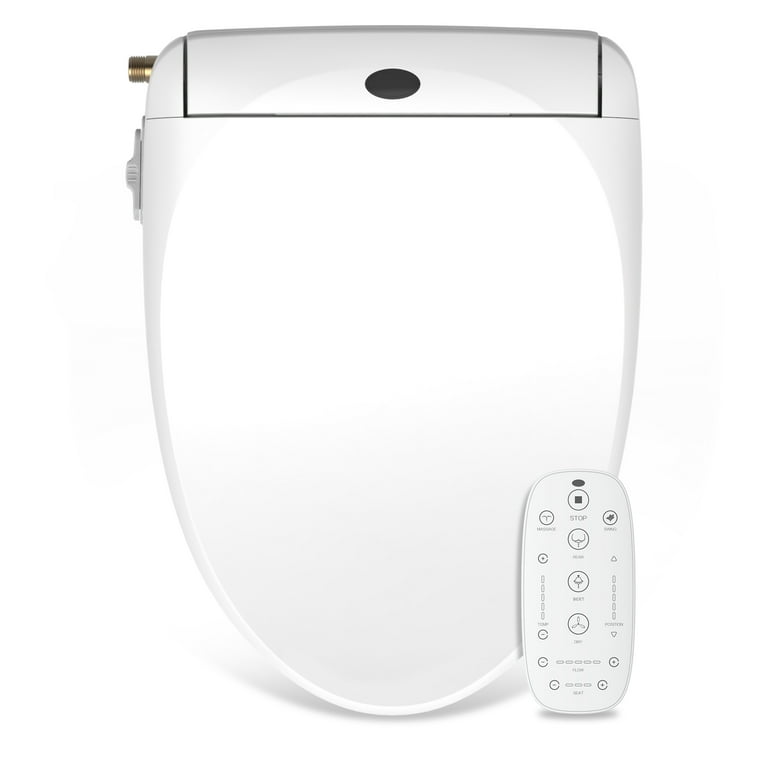The photograph displays a white clamshell-shaped device, strongly resembling an electric bidet toilet seat, positioned against a white backdrop. The device remains closed with a notable oval black insert or sensor at the top center, alongside a protruding gold bolt on the top left. To its side, there is a gray section that includes a button or switch, connected to visible threaded piping. Accompanying the bidet is a small elliptical remote control placed in front, designed with circular operational buttons, including a discernible "stop" button and various other indistinct symbols.